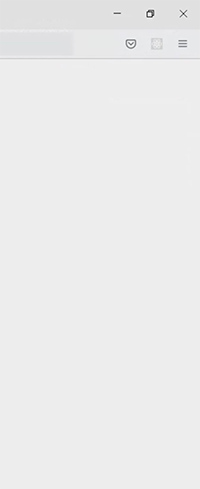This cropped screenshot captures the intricate details of a web browser interface. At the bottom, the page body features a very light gray background, while the very top of the image is adorned with a slightly darker gray. Nestled between these two regions is a medium gray header, seamlessly blending the two shades of gray.

In the topmost header, the top right corner is populated with three dark gray icons arranged from left to right: a minimize icon depicted as a simple minus sign, a maximize icon displayed with two panes stacked one above the other, and a close icon represented by an "X."

Just below this header, situated in the second header, you can glimpse the right side of a medium gray search box on the far left. This search box is followed by a stretch of negative space that leads to a dark gray icon resembling an outlined shield with a small carrot symbol inside. To its right, there resides a light gray square icon featuring a white spirograph pattern, succeeded by a dark gray hamburger menu icon.

Below these elements, a thin medium gray line runs along the bottom of the second header, demarcating it from the light gray body of the page. This section of the page is characterized by open negative space, devoid of any markings or text. Another subtle, almost indistinguishable, light gray line separates the two headers from one another, slightly darker than the top header, yet maintaining the overall grayscale theme of the design.